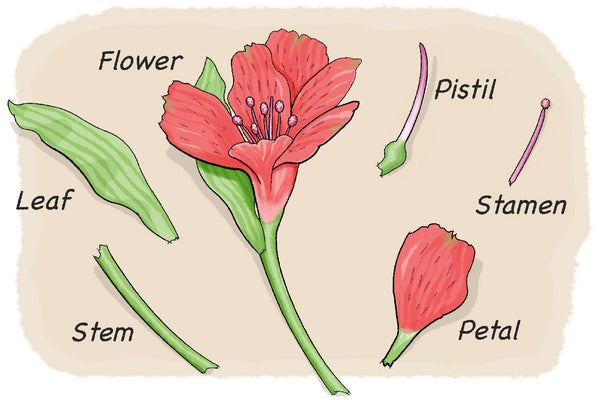The illustration depicts the various parts of a flower against a light tan, beige background with rounded edges. In the center of the image is a cross-section of the flower itself, which features a green stem, green leaves with vertically striped patterns, and six reddish-pink petals. 

The parts are meticulously labeled in black lettering. The central flower is marked with the word "flower" at the top, showing off its seven stamens and pistil. To the left of the flower, the label "leaf" identifies a long, thin green leaf detailed with darker green vertical stripes. Below the leaf, the word "stem" names the slender green support that holds up the flower.

Moving to the right, the word "pistil" labels the key reproductive organ illustrated with a bulbous green base tapering into a white and pink gradient. Further right, "stamen" is used to describe the thin pink filament topped with a small ball. Lastly, beneath that, the word "petal" is paired with the darker pinkish-red petal, showcasing a small green stem.

Each component is clearly illustrated and labeled, ensuring a comprehensive understanding of the flower's anatomy.